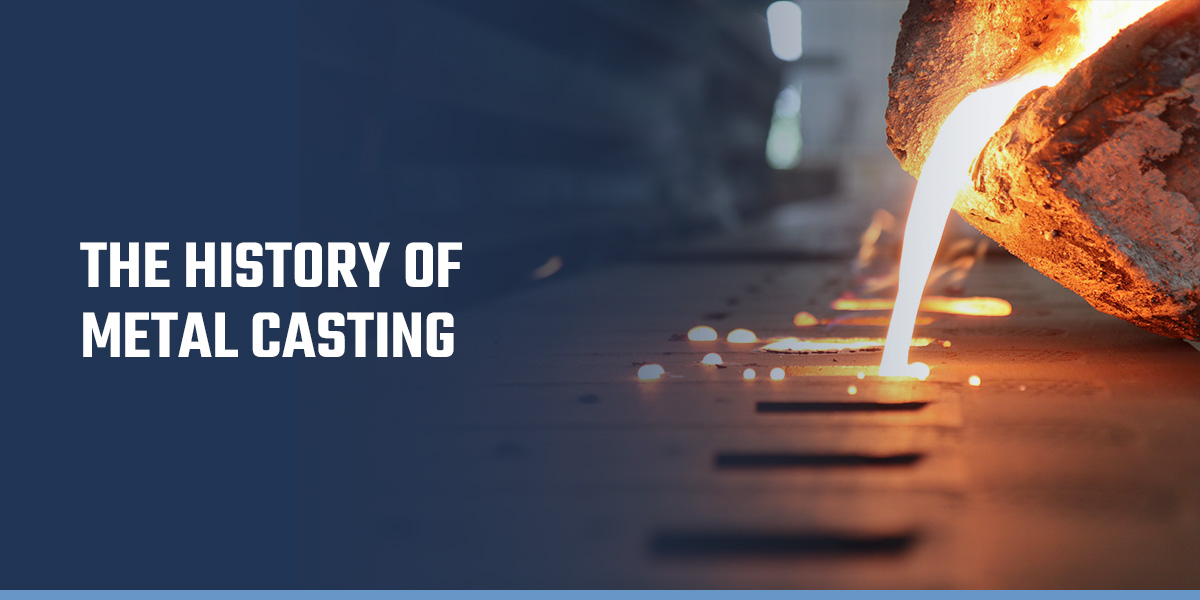This detailed caption synthesizes the descriptions for the image:

The image, resembling an advertisement or textbook illustration, features a poster titled in white Blackletter font, "The History of Metal Casting," on a dark navy blue background that fades into a vivid scene of molten metal casting. The right side of the image dramatically showcases fiery, liquid metal being poured from a glowing red-hot pot into a series of molds, which are arranged on a conveyor belt. These molds appear like they might be forming gold bars, with some filled to overflowing. The molten metal is depicted as intensely bright, akin to the brilliance of the sun, creating droplets that collect below. The background remains indistinct, a blur of dark gray and black with light spots, ensuring that the luminous and dynamic act of metal casting captures and holds the viewer's attention.